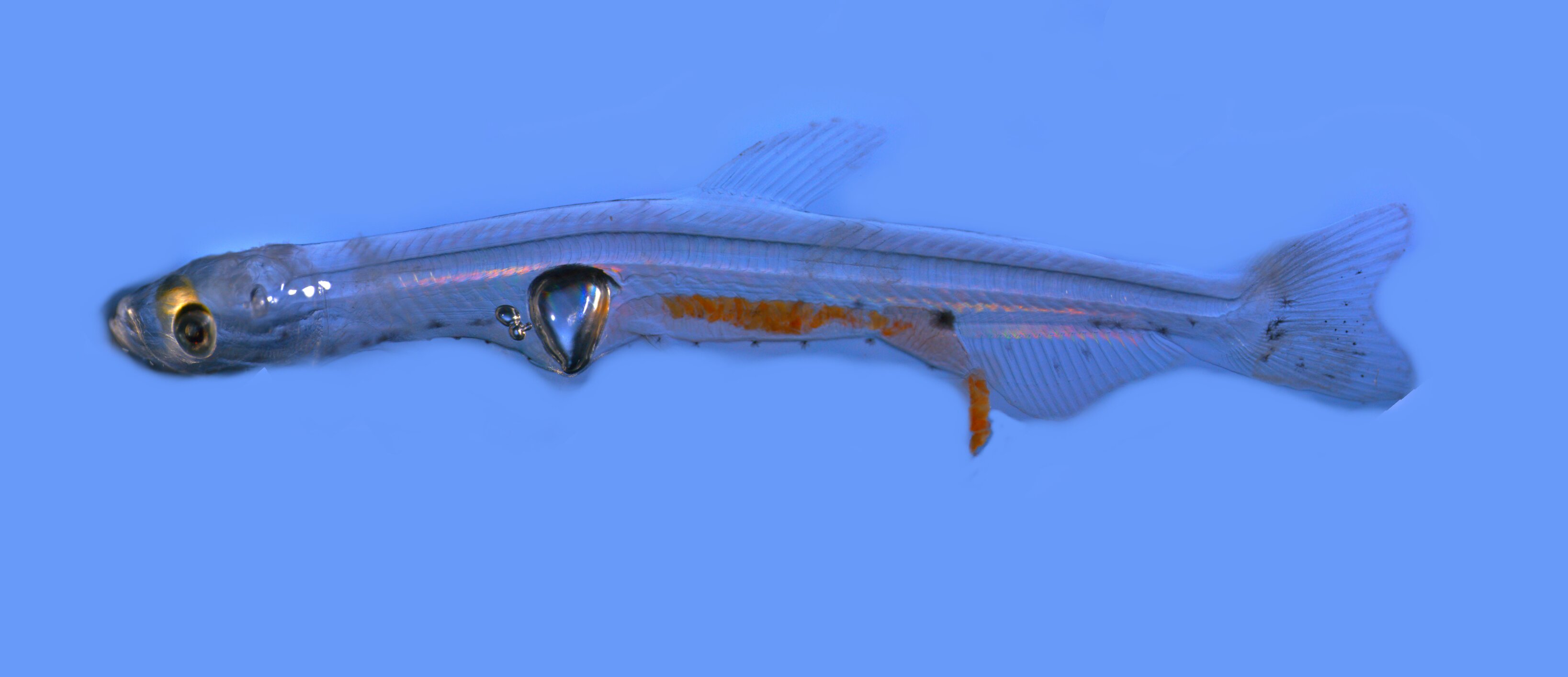The image depicts a long, almost translucent fish against a bright blue background. The fish, which appears to be of microscopic size, displays an array of colors including blue, light blue, orange, black, yellow, and pink. Its scales shimmer with pink hues, while an orange streak runs along the lower portion of its body, contributing to its vibrant appearance. The fish's most striking feature is its large, glowy, gold eye with a yellow circle near it. Its fins include a prominent fin on top and two fins near the back, as well as a distinct left fin that also exhibits a glowing quality. Additionally, you can discern some internal features and a triangular-shaped organ suggesting its reproductive system. The fish extends from the left side of the image, where its circled face is situated, and spans all the way to the right, culminating in its tail. There also appears to be a bubble-like structure near its head, adding to the intricate details of the fish's form.